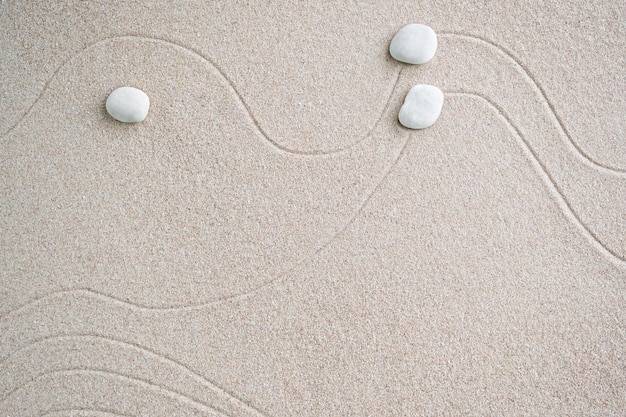The image displays a close-up view of a sandy area with a whitish background speckled with hints of pink. The overall texture resembles fine grains of sand, predominantly tan in color. Spread across the sand are intricate, hand-drawn squiggly and spiral-shaped lines that resemble etched indentations, creating a sense of movement and design. In the image, there are three white pebble-like objects, irregular in shape and scattered at different positions, mainly near the upper left-hand corner and the top area. The lines and pebbles together create a tranquil, almost zen-like composition against the sandy backdrop.